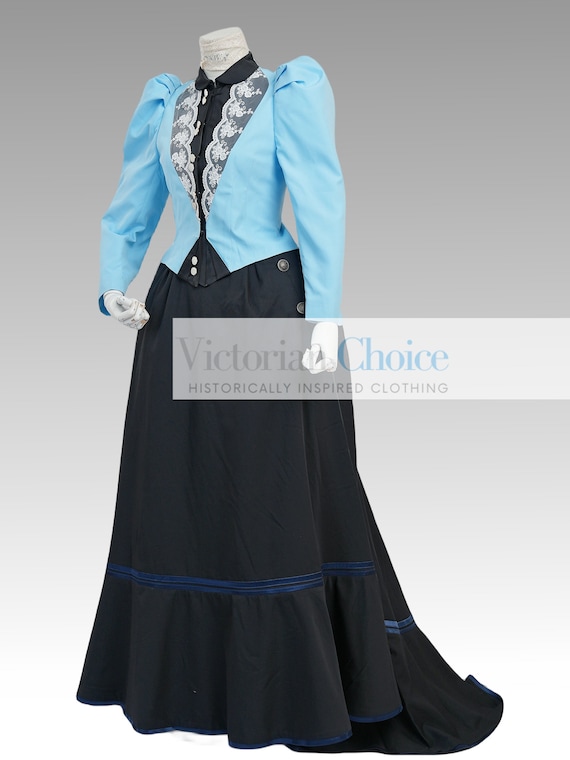This is an image promoting Victoria's Choice, historically inspired clothing. The image features a headless mannequin showcasing an elegant ensemble reminiscent of the Victorian Edwardian era, specifically between the 1890s and 1900s. The centerpiece of the outfit is a light blue jacket adorned with white frilly lace patterns on the lapels and a lace border down the front. The jacket is worn over a flowing black dress that reaches the floor, featuring dark blue trim along the rim and extending into a tail that drags slightly behind. The shoulders of the jacket have a classic puffed design, and it includes subtle details like two white buttons on the side and a small zipper at the bottom. The dress itself is complemented with dark blue accents, including a thick border around the middle and a thinner border at the hem. The mannequin's hands are visible, highlighting how the jacket would fit over someone’s arms. The background fades from gray to white, and across the middle of the image, there is a light grayish strip with a description: "Victoria's Choice, historically inspired clothing," where "Victoria" is written in gray and "Choice" is in light blue.